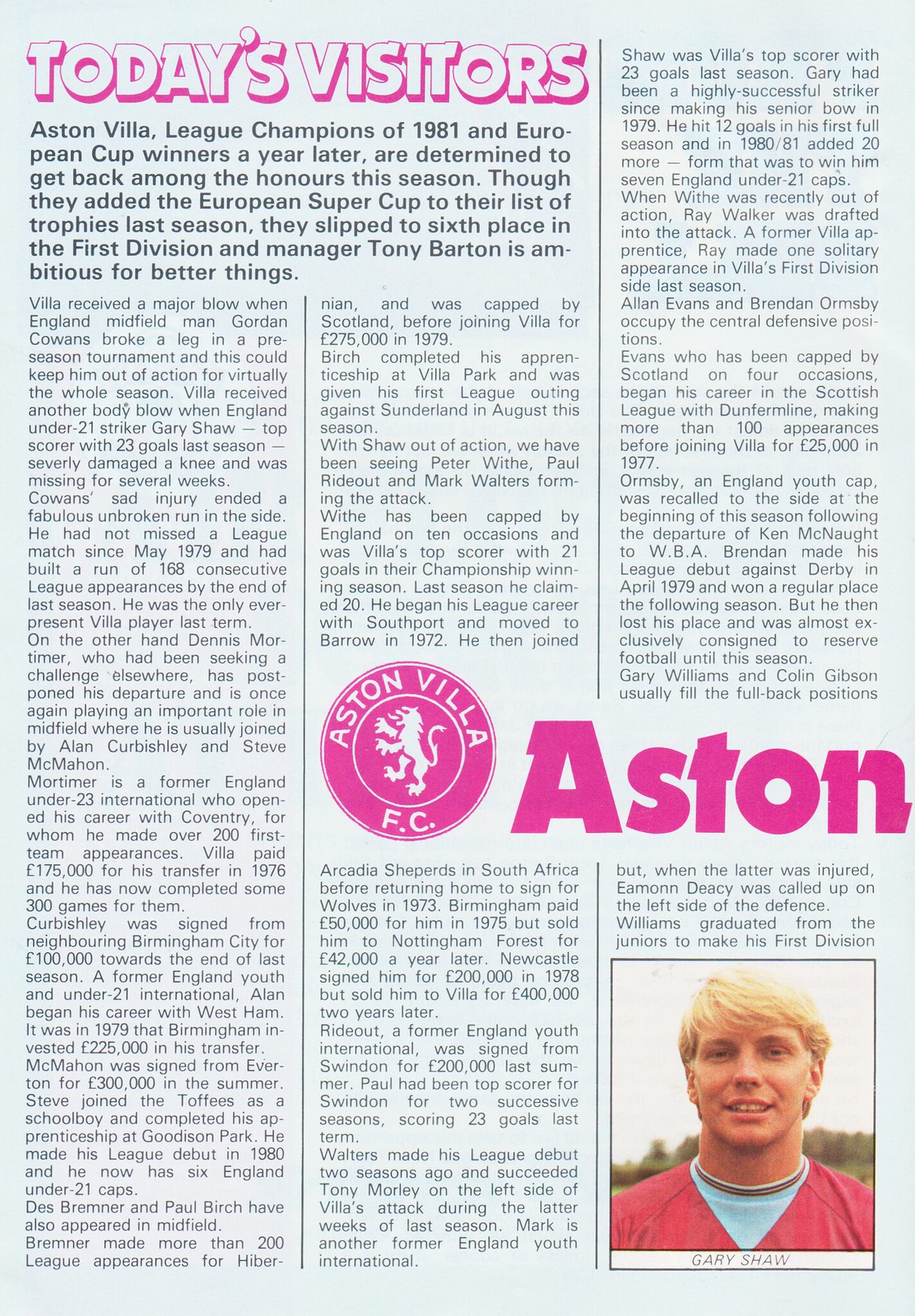The image depicts a newspaper article presented on a light blue background with three vertically separated columns of text, resembling a typical newspaper layout. The title "Today's Visitors" is prominently displayed at the top in white letters with a pink shadowed outline, centered across the top two-thirds of the layout. Beneath the title, a paragraph in black text reads, "Aston Villa League champions of 1981 and European Cup winners a year later are determined to get back among the honors this season. Though they added the European Super Cup to their list of trophies last season, they slipped to sixth place in the first division, and manager Tony Barton is ambitious for better things."

Approximately two-thirds down the layout, spanning the middle and right columns, is a circular logo for Aston Villa FC, featuring a lion in the center and the letters "FC" at the bottom in pink font. Adjacent to the logo, the word "Aston" is displayed in large pink letters. In the bottom right column, there is a photograph of a young man named Gary Shaw, who has blonde hair and is wearing a blue t-shirt under a red sweater.